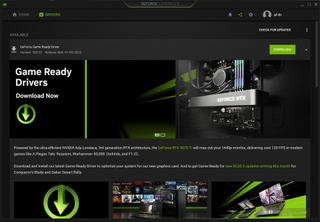The image features a webpage with a predominantly black and very dark grey background, making it challenging to read certain elements. The central, legible portion displays a prominent banner that reads, "Game Ready Drivers, Download Now." To the right of this heading is an intricate image that appears to depict the internal components of a digital device or machine.

The design incorporates several highlighted features in a vivid apple green color, which might suggest a possible, albeit uncertain, association with the technology company Apple. Below the central banner, there is an abundance of tiny, white text on a dark grey background, rendering it nearly indecipherable.

In the bottom left corner of the image, a distinct green circle with a large, downward-facing green arrow is visible, likely serving as an additional download button. This larger button contrasts with a smaller download prompt found above. On the right side of the image, the design includes an open laptop against a green background, completing the technology-themed layout of the page.